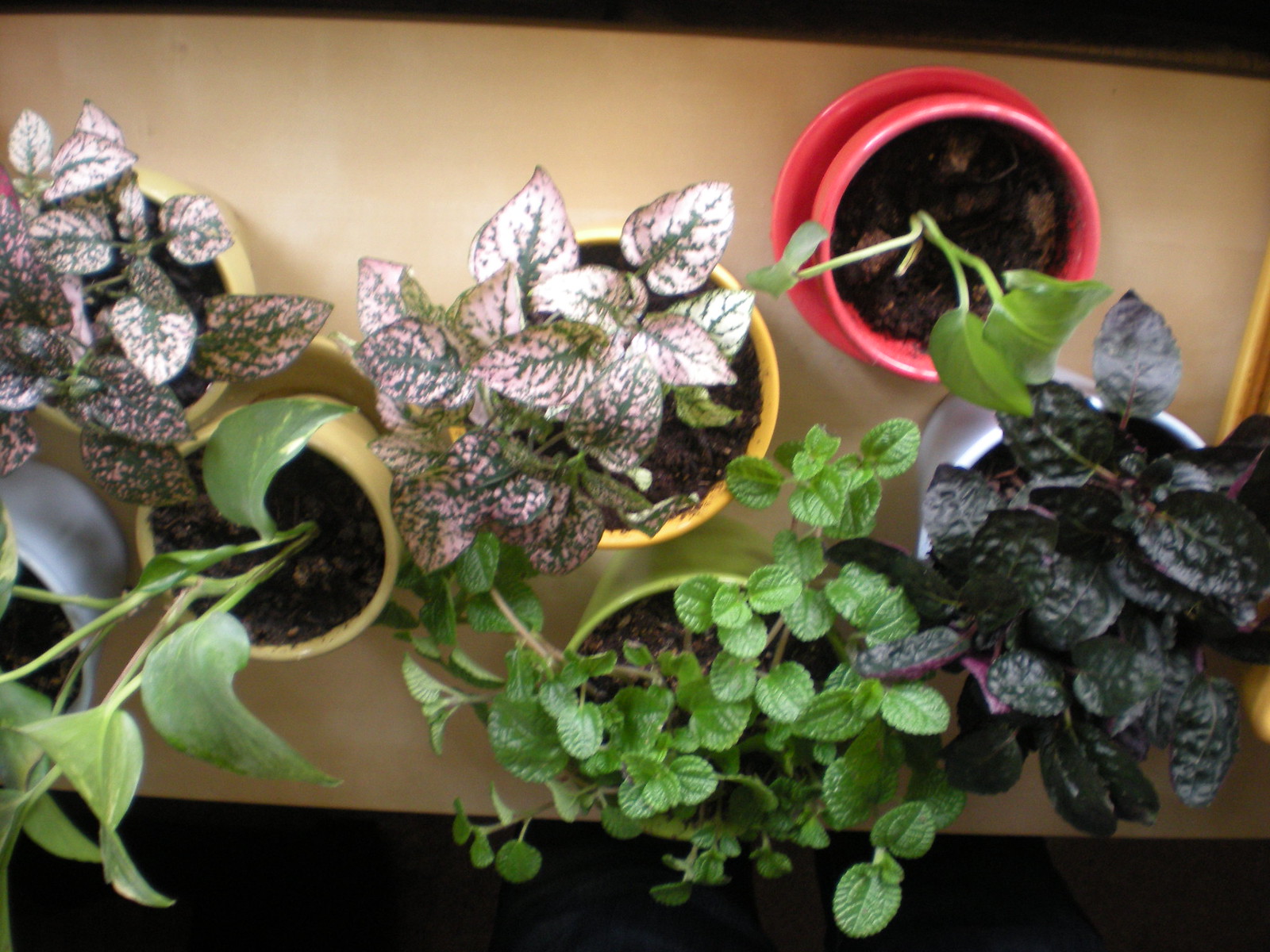This overhead shot captures a diverse collection of young, freshly propagated potted plants resting on a brown table. There are eight small pots, varying in color: three are yellow, with the others being white, red, green, and tan. The sizes of the pots are modest, akin to that of a coffee cup. At the far left is a white pot, followed by two yellow pots, a green pot at the bottom, a red pot at the top right, another white pot at the bottom right, and what seems to be a vibrant yellow object barely visible off to the right.

The plants themselves exhibit a range of leaf colors and shapes. Two of the plants have predominantly green leaves with white variegation. Another features large, curving green leaves, while one has small, sharply defined green leaves. Notably, the plant in the white pot at the bottom right boasts dark, almost black, purplish leaves reminiscent of purple spinach. Additionally, one plant displays green leaves with pink splotches, and another includes golden pothos among its foliage. The sunlight streaming in from the top of the image enhances the visibility of the plants' details. The photo, slightly blurry and taken from a bird's eye view, even captures someone's legs in the frame, emphasizing its casual, almost spontaneous nature.